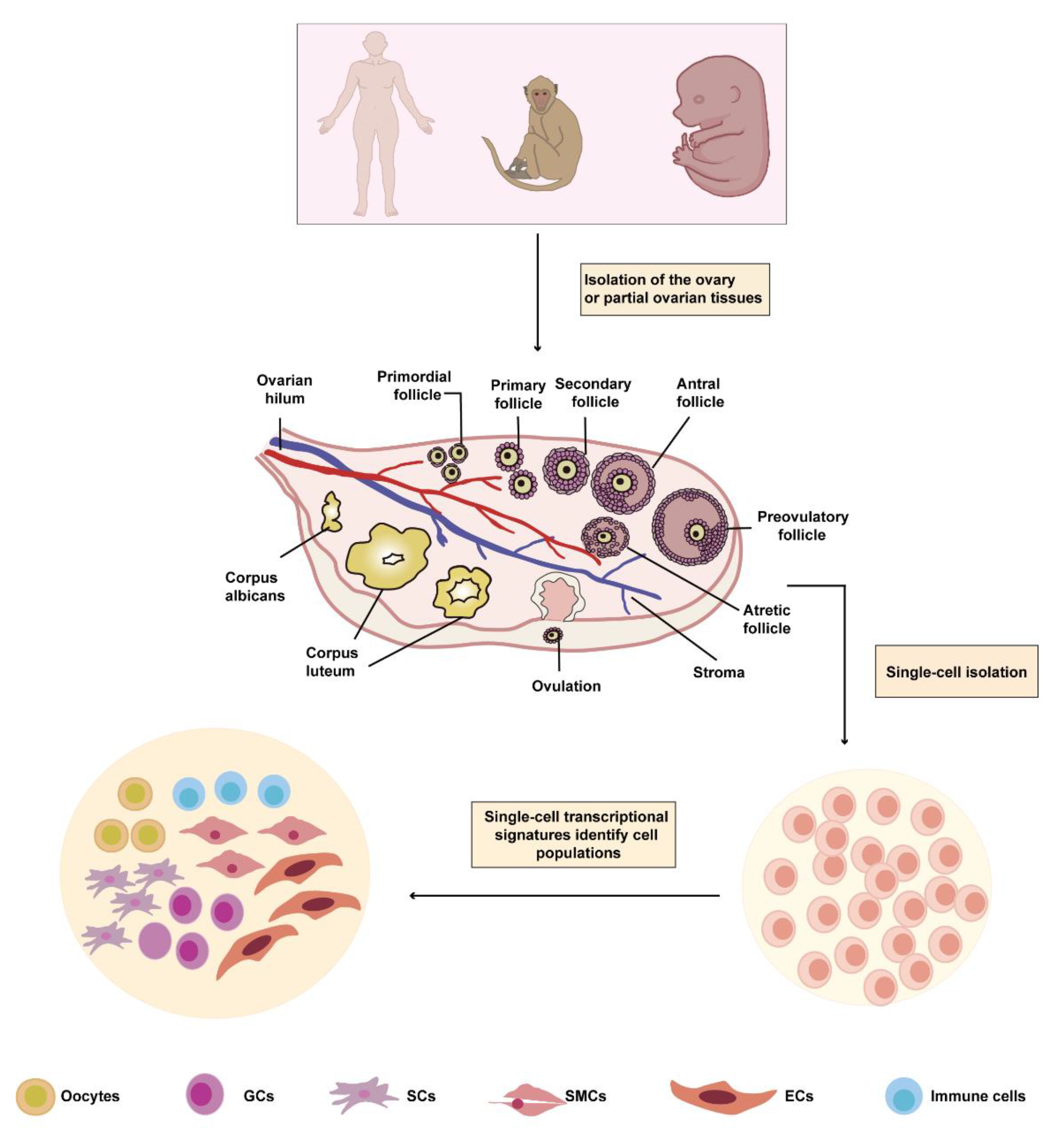The scientific information poster illustrates the isolation of the ovary or partial ovarian tissue, featuring detailed diagrams and labels. At the top, silhouettes of a human, a monkey, and an ambiguous embryo (potentially human or primate) are depicted, indicating comparative studies. Central to the poster is a detailed diagram of an ovary, with labeled parts including the primordial follicle, primary follicle, secondary follicle, atretic follicle, stroma, and the stage of ovulation. The diagram showcases a pink ball filled with smaller, color-coded components, with top-row purplish balls and bottom-row green, flower-shaped forms. Two veins, one blue and one red, run through the center, likely illustrating blood vessels. The lower section of the poster focuses on single-cell transcriptional signatures that identify different cell populations. This area features a chart with very small labels denoting diverse cell types like immune cells, SMCs, SCs, and GCs, represented in pink, blue, and green hues. The colors predominantly used are pink, blue, and purple, enhancing the visual distinction between various cell populations.